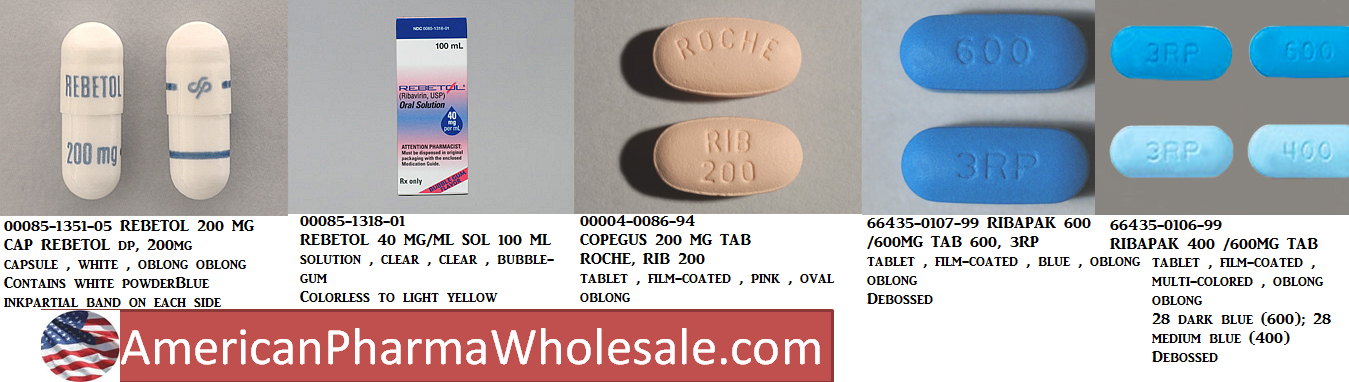In this image, there is a white background with five inset images depicting various types of medication. 

1. The first inset image features a gray box containing two white capsules with blue print labeled "Robitol 200 mg."
   
2. The second inset showcases a white, red, and blue package labeled "Robitol 40 mg."
   
3. The third inset displays two pinkish-brown tablets on a gray background, labeled as "Copagus 200 mg tabs."

4. The fourth inset shows two large, dark blue tablets on a gray background, labeled "Ribopak 600."

5. The fifth inset features four blue pills on a gray background, labeled "Ribopak 400." 

At the bottom of the image, there is a round circle containing an American flag, along with a red block displaying the text "AmericanPharmaWholesale.com" in white print.